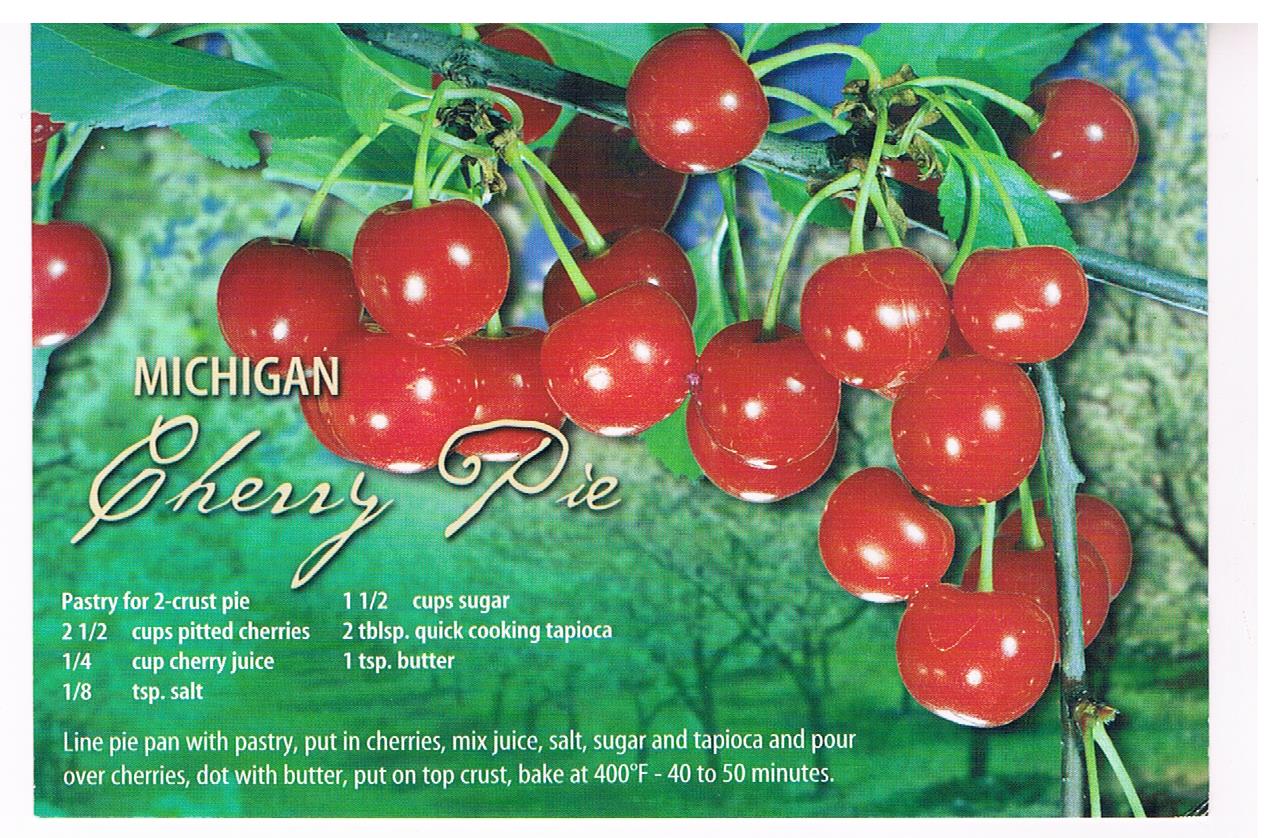The image appears to be a screenshot of a recipe card featuring "Michigan Cherry Pie" prominently in the lower left-hand corner, with a detailed list of ingredients and instructions for making the pie. The recipe includes ingredients such as peanut cherries, cherry juice, salt, sugar, quick-cooking tapioca, and butter, as well as pastry for a two-crust pie. In the upper right-hand corner, there is an illustration of a vine with a bundle of cherry tomatoes, and the background showcases what looks like an orchard or vineyard with green trees, grass, and a clear blue sky. The scene suggests a picturesque countryside setting where cherries and possibly other fruits or vegetables are grown. This detailed depiction aligns with the theme of a cherry-centric recipe, highlighting the fresh, natural ingredients used in the pie.